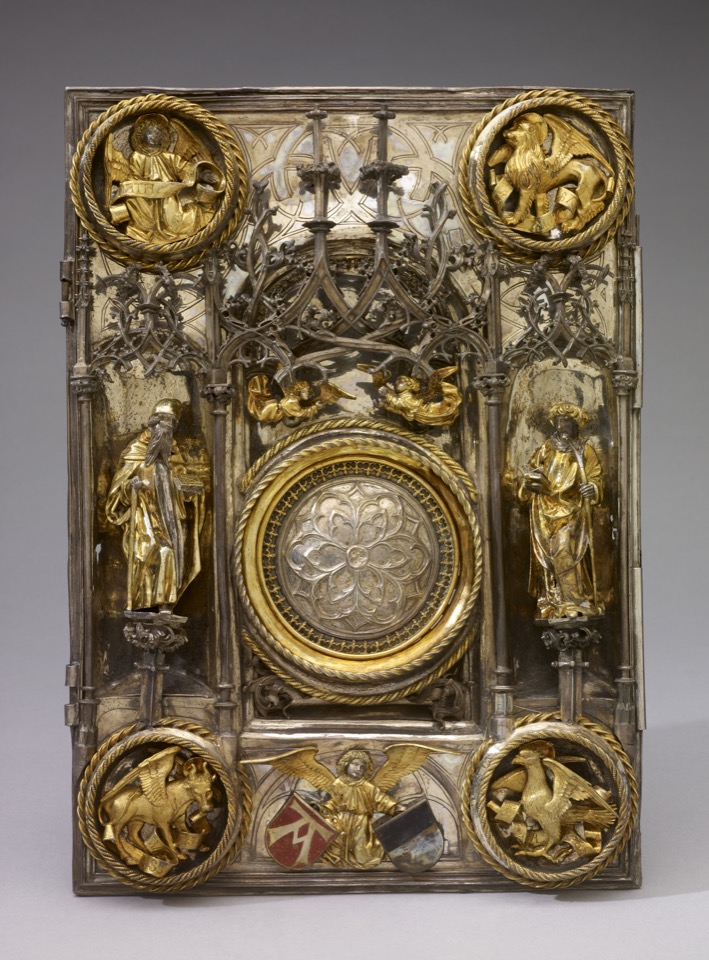The image depicts an intricately adorned, antique book cover set against a gray background, showcasing a masterpiece of ornate metalwork in various tones of gold, brass, silver, and bronze. The cover, likely a symbolic or ceremonial door, features religious and mythical figures in detailed relief. At each of the four corners are circular medallions encased in brass rope, depicting an angel with a banner (top left), a winged lion in profile (top right), a winged goat (bottom left), and a bird with its wings spread wide (bottom right). Central to the design is a silver, circular medallion with an ornate, raised rose carving, surrounded by several rings of differing textures. Bookending the medallion are two religious figures in long robes, each standing on podiums, and above it are two raised candelabrum-like structures. The spaces between the corner medallions on the left and right edges contain smaller pairs of robed figures, while an angel graces the bottom center of the composition. The overall style of the cover is photographic realism, capturing the luxurious and elaborate aesthetic of the piece.